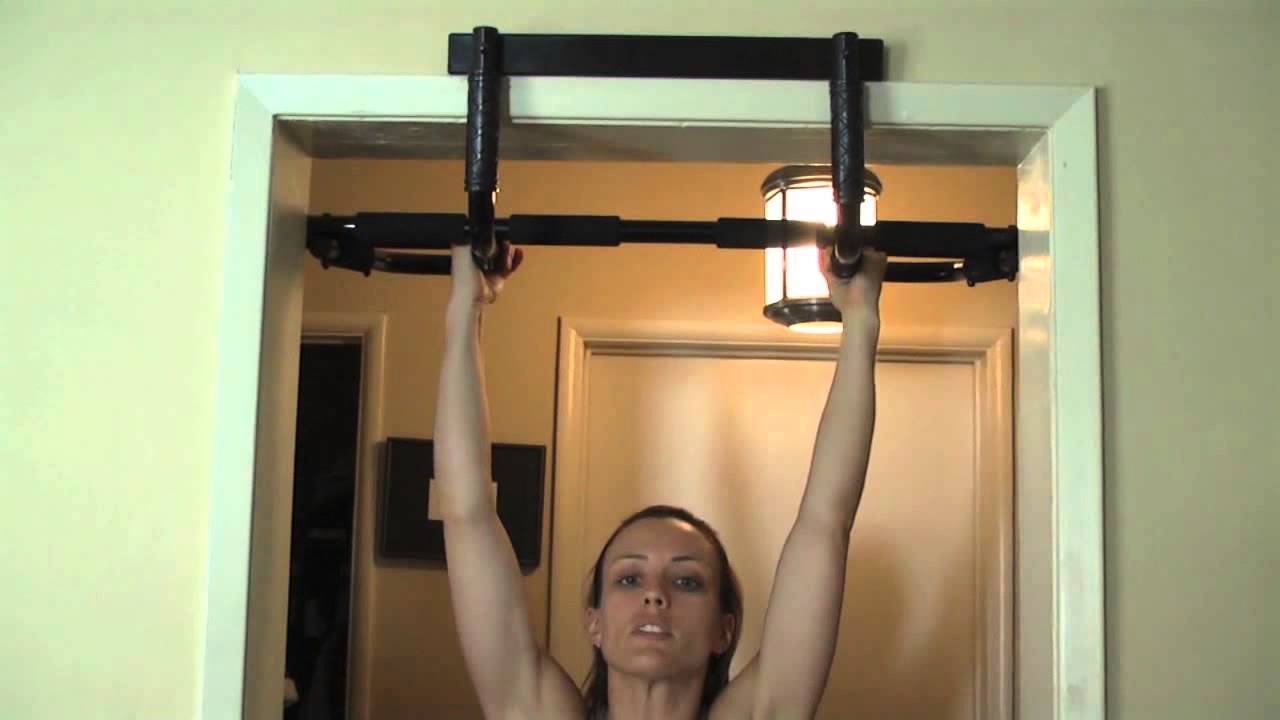In a realistic-looking photograph with a wide horizontal rectangle frame, the image centers on the upper half of a white door frame, set against light beige walls. A black pull-up bar is attached to the door frame, which is the focal point of the scene. Hanging from this pull-up bar is a white woman with dark hair, captured from the shoulders up. Her arms are fully extended, grasping the handles, and she appears to be in the lower position of a pull-up. Her face is slightly tilted upwards, and she is looking directly at the person taking the photograph, with her mouth slightly open, as if preparing to pull herself up. 

In the background, there's a hallway illuminated by a ceiling light, casting a warm yellow glow. The hallway features a white door and an open door frame to the left that leads into a dark space. Additionally, a small rectangular photograph and a plaque can be seen hanging on the walls between the doors. The setup suggests a moment of pause and effort as she engages with the exercise equipment.